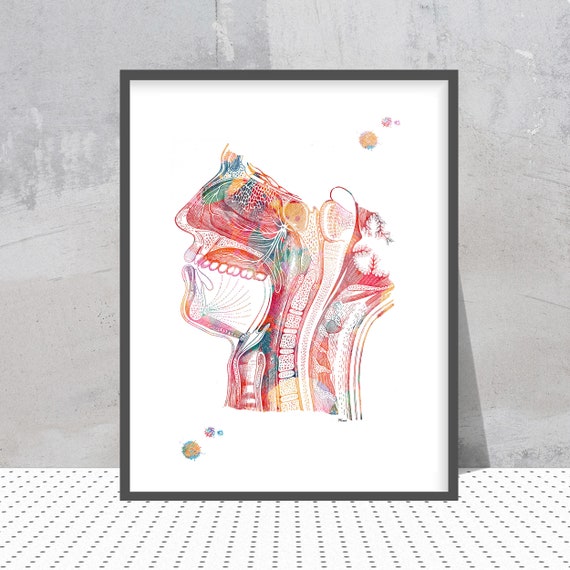This image features a framed artwork placed against a grey concrete wall on a textured, polka-dotted tile floor, predominantly white with black dots. The black-framed print offers a colorful and intricate cross section of a human head in a side profile view, detailing the internal structures from the eyes to the neck. The artwork is bursting with a blend of vivid colors—red, green, yellow, blue, and orange—seamlessly merging into one another in an abstract and aesthetically pleasing manner, with some paint splatters for added artistic effect. The depiction reveals parts of the spine, olfactory system, and the mouth, including the top row of teeth and tongue, although the level of detail appears somewhat stylized or artificially generated, as certain anatomical elements are either missing or inaccurately represented. The print itself is laid out on a simple white background, creating a stark, striking contrast with the black frame and the colorful centerpiece.